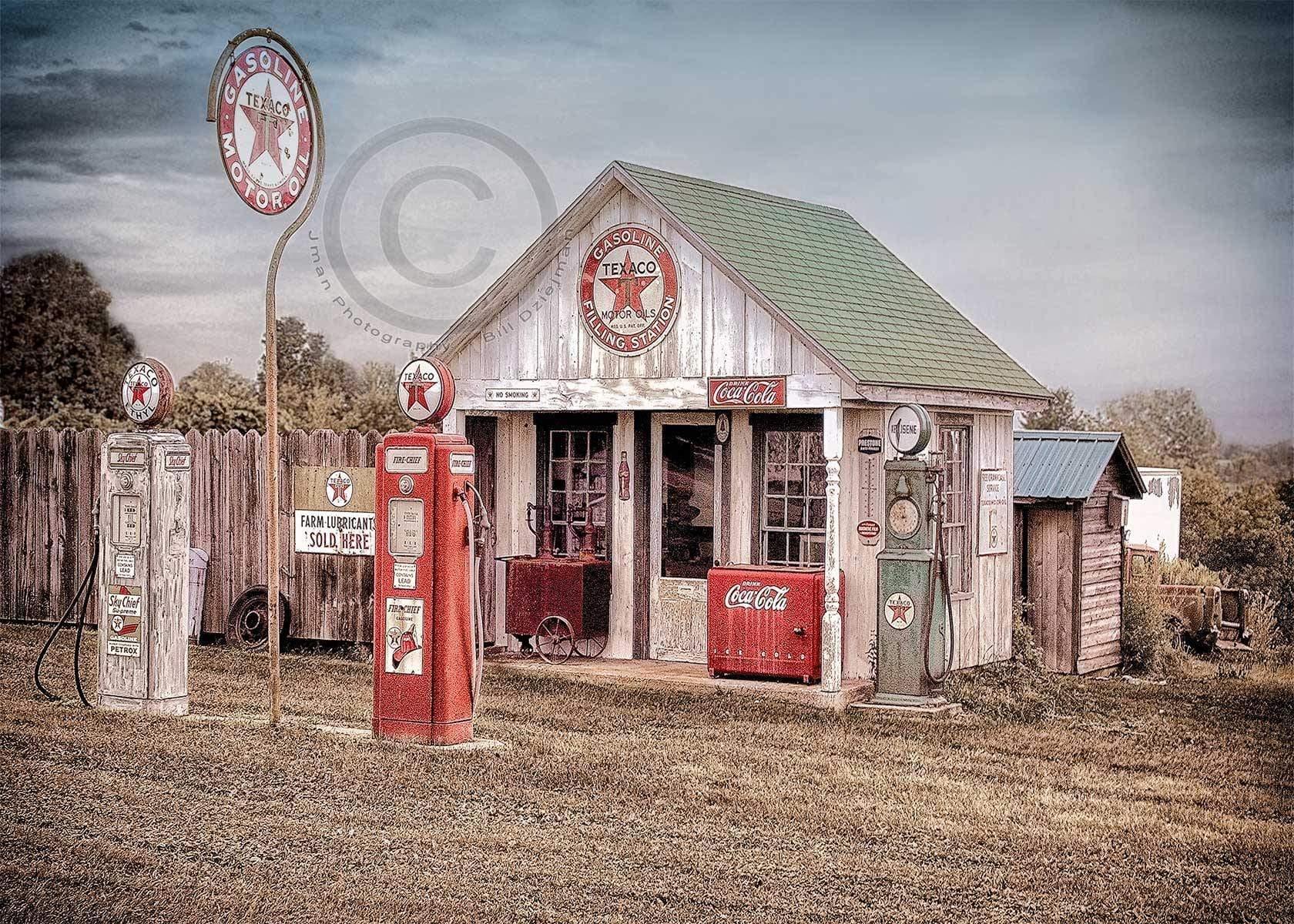This is a highly detailed image of a vintage Texaco gas station, evoking nostalgia with its classic design and rustic elements. The station, constructed with a small house-shaped structure, features a pitched green roof and wooden siding, giving it an old-time feel. Prominently displayed on the front is the iconic Texaco star logo, along with signage that reads "Texaco Gasoline Filling Station" and "Texaco Motor Oils."

Two vintage-style gas pumps stand in front of the station, one in red and another in weathered wood and white, both bearing the classic Texaco star. A third kerosene pump, colored green, is located to the right side of the building. Between the pumps is a large red and white Texaco gasoline motor oil sign.

Adding to the charm, a vintage Coca-Cola sign hangs under the awning, accompanied by an old Coca-Cola ice chest on the small porch—ready to offer a refreshing drink. The surrounding area features dirt and patches of grass, and the cleanliness of the scene stands out. There is a black fence running alongside the backdrop, with trees visible beyond it under a gray, somewhat dark sky. 

This evocative image has been captured beautifully in color by J-Man Photography, with a watermark reading "J-Man Photography" and the name "Bill Dziejman" emblazoned across the center. This iconic snapshot not only captures a bygone era but also immortalizes the care and craftsmanship of early 20th-century Americana.